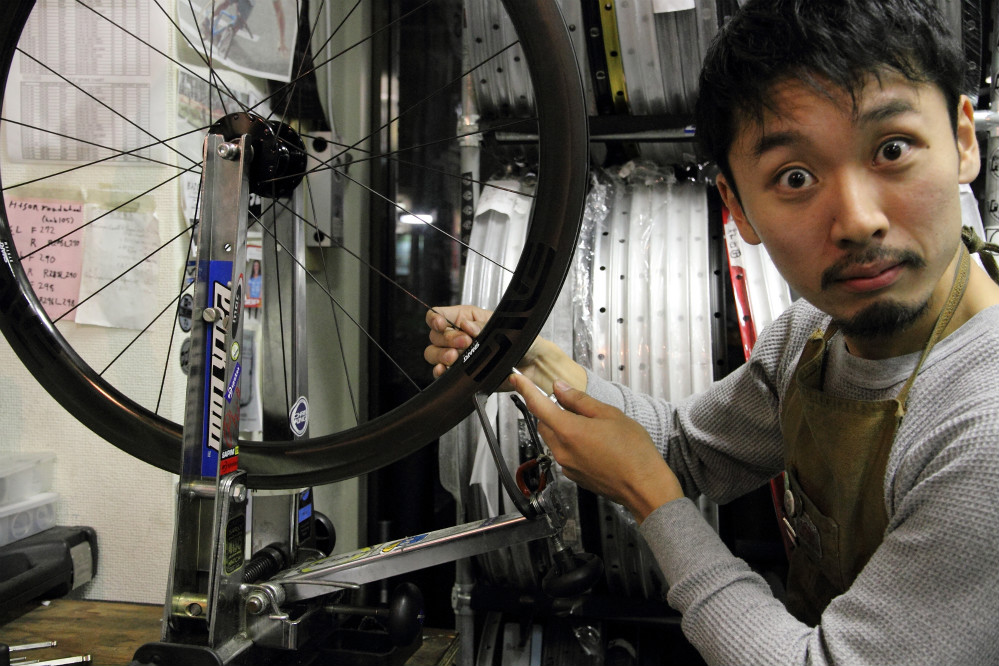In this image, a man, likely of Asian descent, is diligently working in a high-end bike repair shop. He is focused on a bicycle wheel mounted on a truing stand fixed to a table, fine-tuning the spokes with his right hand while his left hand supports his work. The man sports a gray, long-sleeved, waffle-weave shirt and an apron, appropriate for a repair technician. His facial expression is humorous, with eyes wide open in an exaggerated manner, attempting to look funny. His appearance is characterized by a mustache and a small goatee. The background reveals a well-equipped bike shop, showcasing a variety of rims in different shapes and colors, suggesting a sophisticated inventory. Behind him, a bulletin board filled with various notes and a photograph—details of which are unclear—adds a touch of personal touch to the workspace.